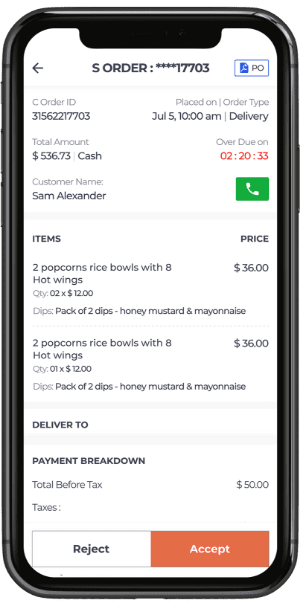The image shows a smartphone screen displaying an order summary interface. 

- At the top left corner, there's a back arrow icon.
- The top center reads "ORDER ORDER" in all capital letters.
- Below that, there is a code "**** 17703" alongside a blue rectangle labeled "PO."
- In a lighter font, the text "See Order ID Placed On | Order Type" is shown, followed by the relevant numbers.
- The "Total Amount" is displayed, with an "Overdue On" section to the right, showing the overdue date in red and the overdue amount in black.
- Below this information, the customer's name is shown next to a small green box featuring a phone icon.
- Further down, the screen lists ordered items on the left, with their corresponding prices on the right.
- The next line reads "Delivered To," followed by "Payment Breakdown," and then "Total Before Tax" with a listed amount of $50.
- The "Taxes" section is present but empty.
- At the bottom, there are two rectangular buttons: one labeled "Reject" and the other "Accept."

This visually detailed description provides a comprehensive overview of the smartphone screen's order summary.